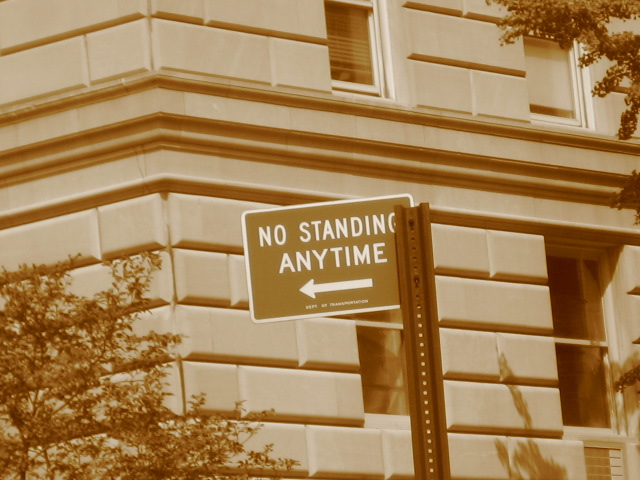The image depicts a "No Standing Any Time" street sign in front of a tall, light-colored building with large, rectangular stone bricks. The sign features a dark background with a white border, and white capital letters with a left-pointing arrow. Beneath the arrow, there are very tiny letters, likely indicating the Department of Transportation. The supporting post for the sign has distinct holes through it, similar to typical street sign bars, and only the top portion is visible. The picture appears to have a sepia tint, giving it a light brownish-orange hue, which affects the color of the sign and surroundings. In the background, the building has visible windows, some with open blinds and some with closed, adding to the aged and slightly weathered appearance. The scene is framed by the tops of trees on both the left and right sides of the image, viewed from a higher vantage point.